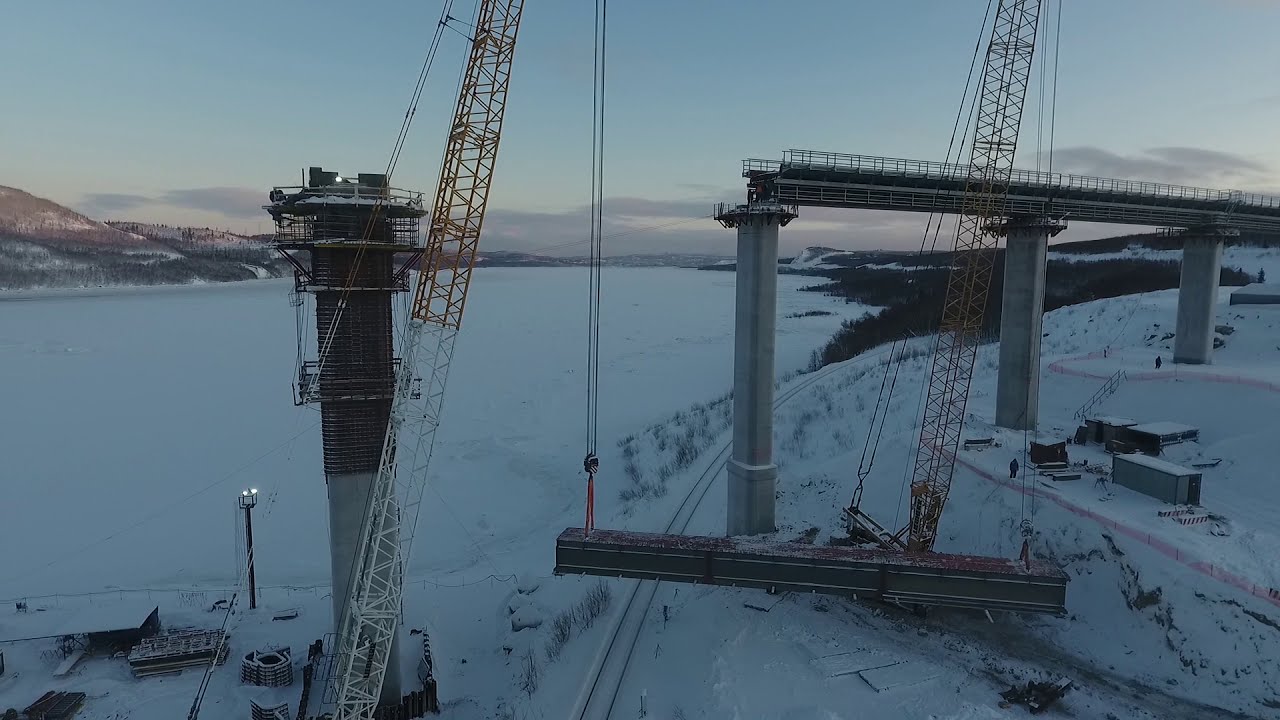This photograph captures a vast and snowy landscape, possibly taken early in the morning or just before sunset, lending a soft light to the scene. The focal point is a large construction site where a bridge is being built over a frozen or snow-covered body of water. Dominating the site are three to four massive concrete pillars, some reaching at least 50 feet high, with partially constructed bridge sections resting atop them. Two large yellow and white cranes are actively lifting building materials, with wires hanging from them, emphasizing the scale of the construction work. Surrounding the site is a stark white terrain, interspersed with some trees and bushes, and in the background, hazy blue sky and distant hills or mountains complete the serene yet industrious vista. No people are visible, enhancing the focus on the monumental infrastructure taking shape amidst the wintery setting.